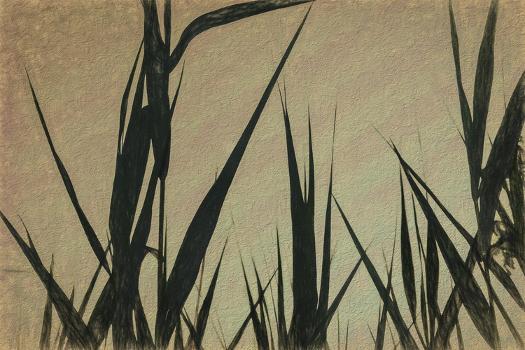This is a large rectangular painting, capturing a scene of tall, thin grass blades silhouetted against a tannish brown background. The blades of grass, rendered in dark green hues that almost appear black in the setting sun, are arranged in several distinct clusters, each pointing in different directions to give a sense of natural disorder. At the base of some clusters, tiny brushstrokes suggest smaller pieces of grass sprouting up. The background transitions into a grayish sky, evoking the moments just before sunset, when the sky is darkening and colors are fading into silhouettes. From a bottom-up perspective, emphasizing the tallness of the grass, a larger central blade forks off in the middle, flanked by slightly smaller leaves on both sides, some extending diagonally and others straight up. The painting captures the essence of a random field at dusk, with light shading adding depth and texture to the dark green and black forms of the grass blades.